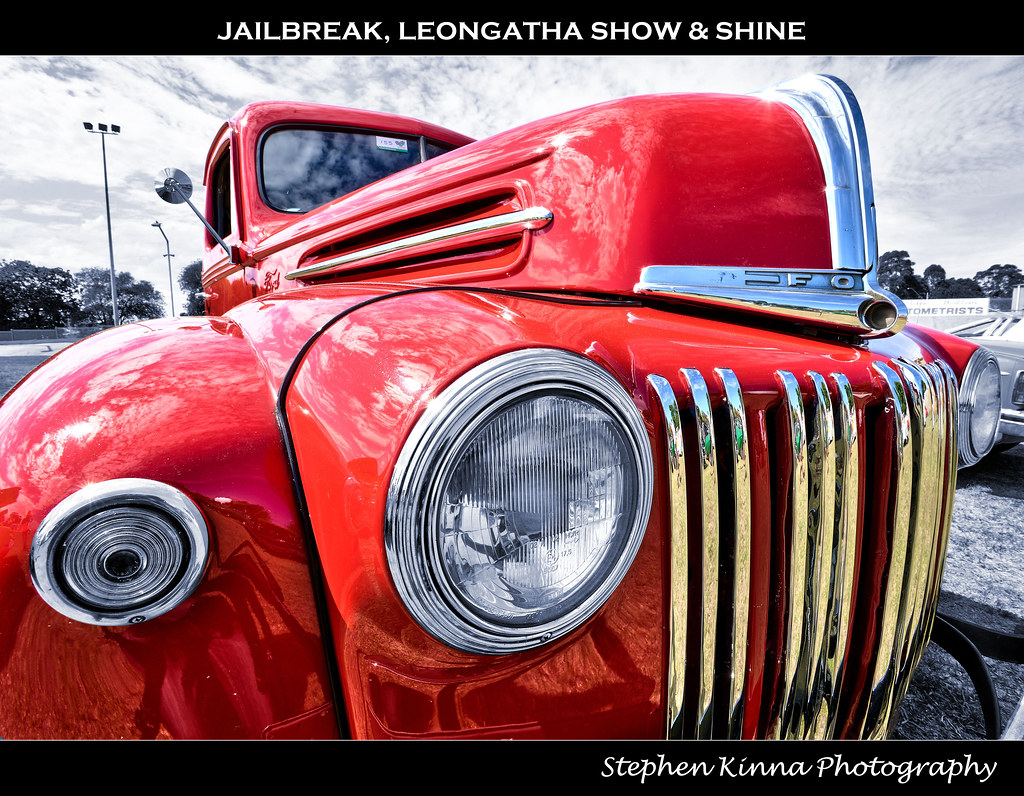This highly detailed and stylized photograph captures a vibrant cherry red classic Ford pickup truck in impeccable, fully restored condition. The truck features large round headlights encircled by polished chrome, and a prominent, vertical chrome grille with multiple vertical slats. The reflective chrome accents on the hood and around the headlights add to the vehicle's striking appearance. The vibrant red paint appears fresh and glossy, adding to the truck's aesthetic appeal.

The background has a grayscaled effect with a subtle bluish tint, enhancing the truck's vivid red color. In the background, there are stadium lights to the left, suggesting the scene might be a baseball field with trees and other classic cars parked in the vicinity. Across the top of the image is a black bar with white text in the center that reads "Jailbreak, Leong at the Gotha Show and Shine." In the bottom right corner, cursive text reads "Stephen Kina Photography," attributing the photograph to its creator.